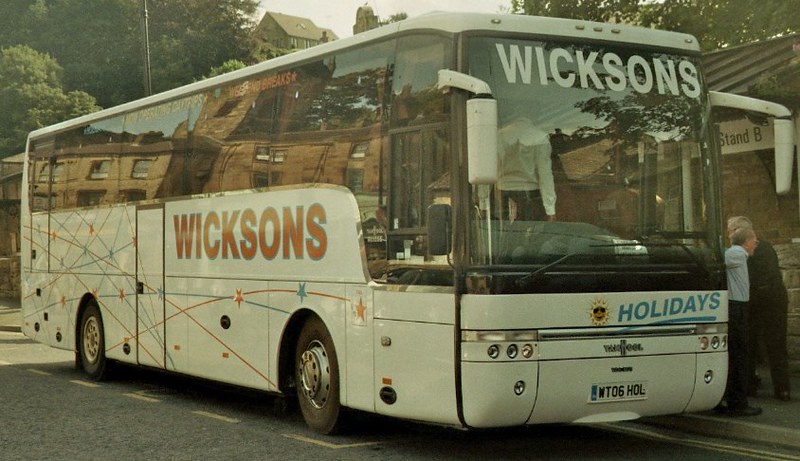The image depicts an older, slightly grainy photograph of a parked Wixens-branded bus, identifiable by the name "Wixens" displayed on both the front and left side of the vehicle. The bus itself is predominantly white, with blue and orange lines running across it, complemented by matching blue and orange stars. The lower two-thirds of the bus showcase these decorative elements, while the upper portion features heavily tinted windows.

Central at the front, just below the windshield, is an inscription reading "holidays" accompanied by a picture of a sun, and below that, the bus’s plate number is visible. Inside the bus, a man is seen wearing a white T-shirt and a white long-sleeve button-up shirt paired with trousers.

Outside the bus, on the right side, there are two older men. One is wearing a blue button-up shirt and trousers, and the other, who is also wearing glasses, is dressed in a black shirt, black pants, and black shoes. The photograph's background showcases some greenery with trees and their lush green leaves, as well as the roof of a building and a bit of gray sky, all of which contribute to the scene’s slightly nostalgic ambiance suggestive of a 70s or 80s timeframe.